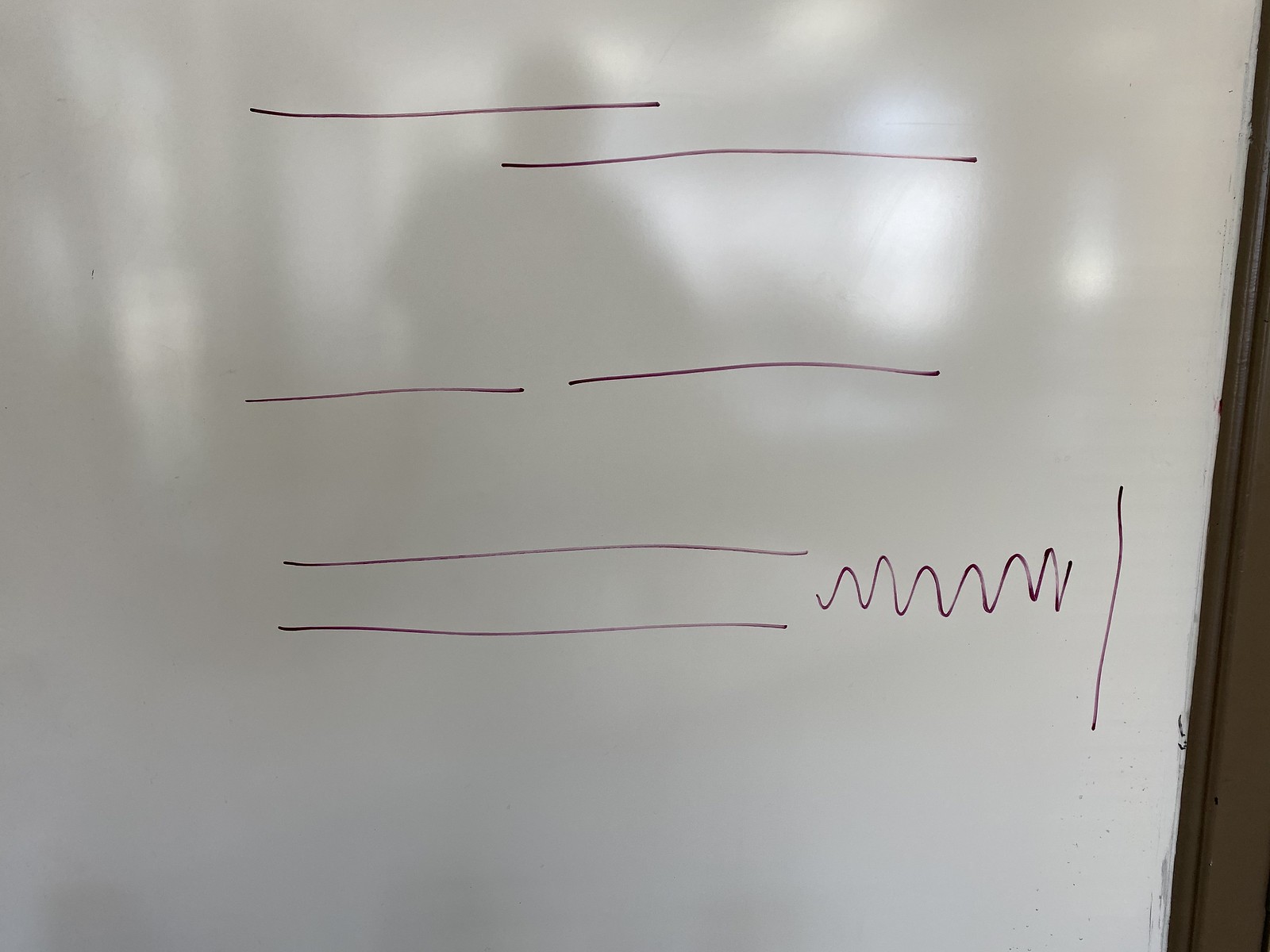In the photograph, a large whiteboard is prominently displayed, reflecting the brightness of a summer day. The whiteboard's surface captures faint reflections, hinting at the presence of open windows in a possible school or office setting. On the right side of the image, wooden paneling is visible, extending to an adjacent open window, pouring natural light into the room.

The whiteboard itself, devoid of any clear writing, features random markings made with a purple marker. At the top of the board, a single purple line extends horizontally. Approximately two or three inches below it, another line appears, partially overlapping the first. Farther down, a pair of parallel lines are spaced several inches apart, hinting at the board's substantial size. Below these, another set of parallel lines is visible, accompanied by a squiggly line with six distinct humps. A solitary vertical line stands isolated among the chaotic array of marks.

In the middle of the whiteboard, the faint shadow of a person—likely the photographer—adds a human element to the scene. To the right, a column is partially visible, contributing to the architectural features of the room. On the left side of the image, a bulletin board adorned with pinned papers further suggests the setting might be a school, completing the observational details of this photo.